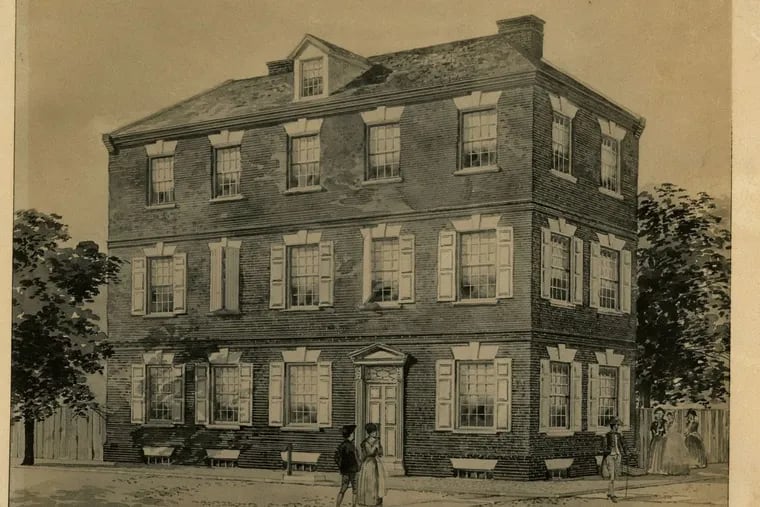The image appears to be a very detailed, black-and-white illustration, possibly a painting, depicting a grand, three-story brick building from the 1700s, possibly set in a colonial French city. The primary focus is the ornate building, characterized by its numerous windows and elaborate design. The front façade of the building features 15 windows, including a dormer window on the roof, and there are six windows on the visible side end. Most windows are adorned with shutters and ornate designs above them. The ground level includes a door in place of one of the windows.

The building has numerous chimneys, indicating multiple fireplaces, which were essential for heating during that period. There are also people walking around dressed in 18th-century French attire, with men wearing tight high pants, long-tailed jackets, sailor-style hats, and carrying canes. Women are also present, enhancing the historical context. The scene includes trees flanking each side of the building and a light-colored sky with visible fences, suggesting an urban setting. The illustration is printed on yellowed paper, showing its age, and is almost photorealistic in its pen-like detailing, emphasizing the building's intricate architecture and historical significance.